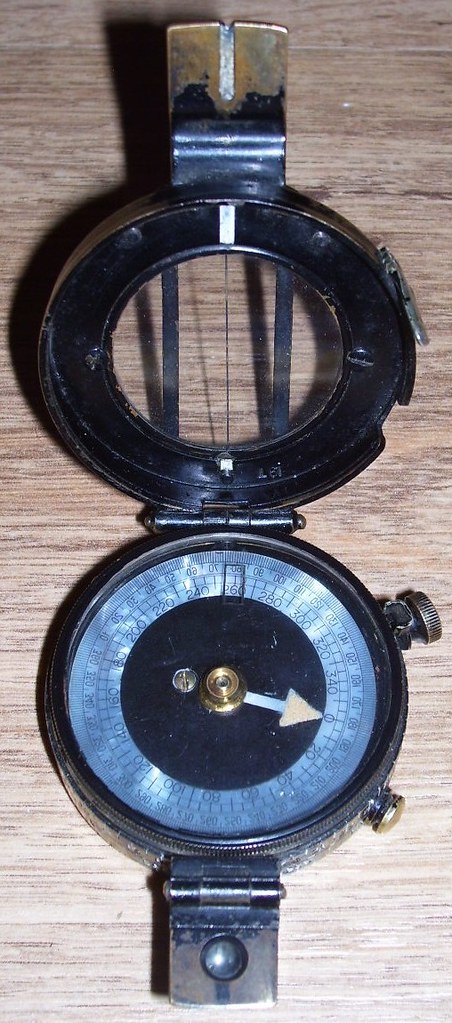This photograph features a circular instrument closely resembling a watch but distinctly not one, appearing more akin to a compass or barometric device. The dial is marked with numerical increments from 0 to 360 degrees, featuring every 20-degree increment. The numbers run sequentially around the dial: 0, 20, 40, 60, 80, continuing through 320, 340, and then returning to 0. A white hand, extending from a central brass fitting, forms an arrow with a triangular tip, demarcating readings on the dial.

The inner circle of the face is a solid black, contrasting with the outer edge, which has a metallic finish with a subtle blue tint. The side of the device showcases a couple of buttons, one of which appears to be a winding knob. A circular faceplate with a hinged clasp is shown in an open position, protruding from the bottom half of the device.

The entire instrument rests on a piece of wood, oriented so that the wood grain runs horizontally across the image. The frame and body of the device are black metal, while the clasp's exposed metal exhibits a brass or bronze hue. A vertical line is drawn across the glass surface, likely intended for aligning the compass, while two external metal bars across the glass serve as protective features.